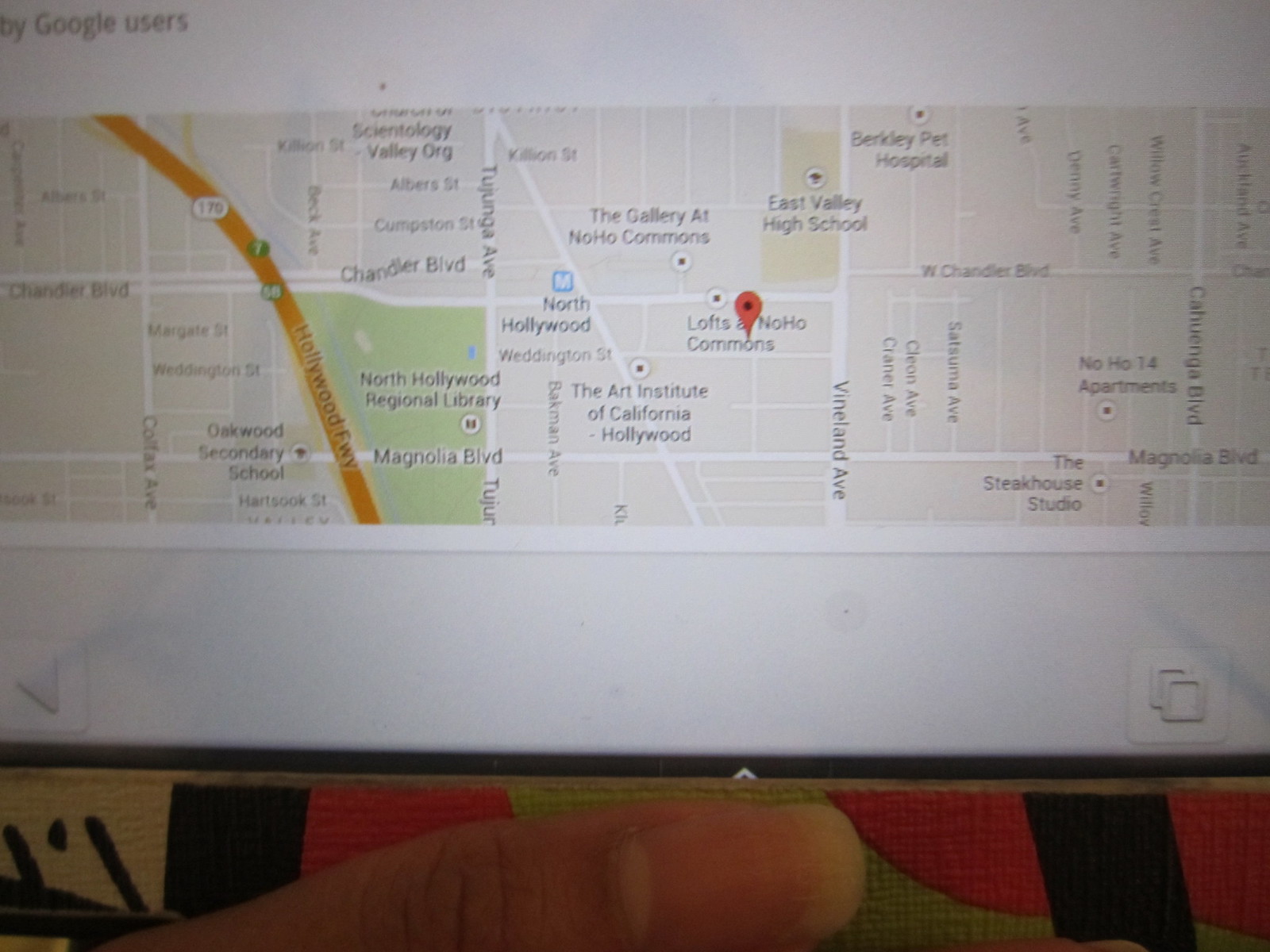The image depicts a blurred photograph of a digital screen, possibly a smartphone or a computer, displaying a map. Central to the map is a prominent red location marker, indicating "Lofts" and "NoHo Commons." The interface at the upper-left corner attributes the map to Google Users. The map also highlights several other areas, including North Hollywood, The Art Institute of California - Hollywood, East Valley High School, The Steakhouse Shallo, Chandler Boulevard, and Magnolia Boulevard. A distinctive yellow line marked "170" can also be seen, likely representing a highway. The device capturing the image is held over a designed placemat, with a visible thumb at the bottom, hinting at the person's grip on the device. Despite the overall blurriness, these key details remain discernible.